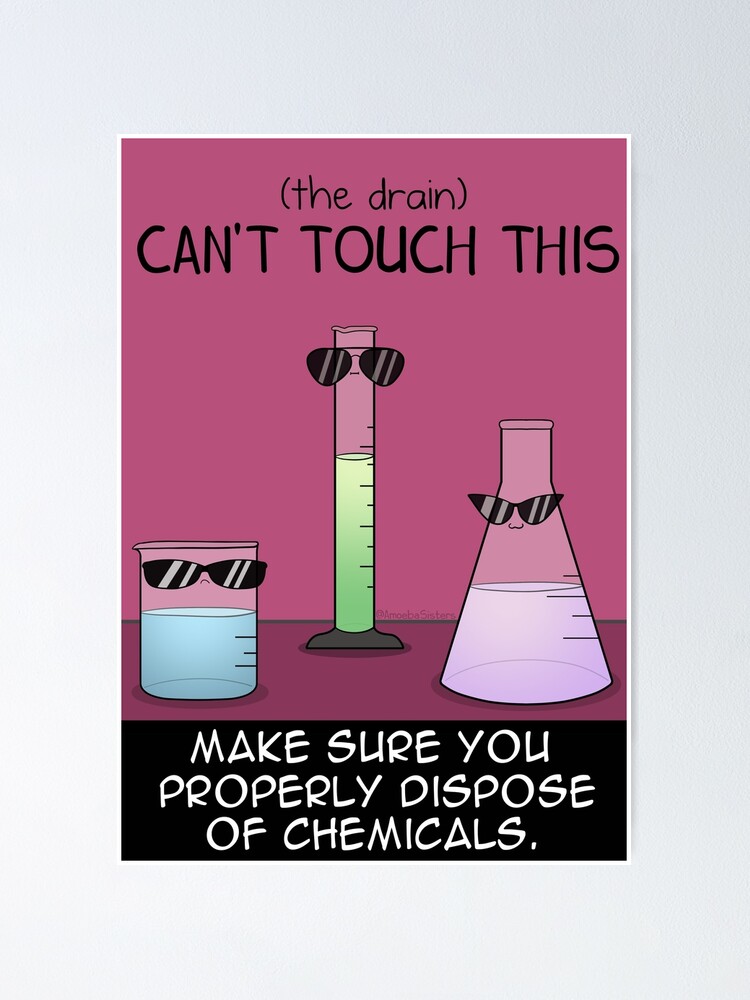A vibrant, cartoon-style poster intended for chemistry classrooms or labs features a playful yet informative message about proper chemical disposal. The poster has a purple to plum gradient background and showcases three character-like laboratory items: a tall, cylindrical beaker with blue liquid, a test tube with green liquid, and a flask with a conical base containing purple liquid. Each character sports sunglasses and a cute anime-style mouth, adding a whimsical touch. The top of the poster displays a catchy headline in a hand-drawn font: "(the drain)" in lowercase and parentheses, followed by "CAN'T TOUCH THIS" in bold, uppercase letters, reminiscent of the MC Hammer lyric. At the bottom, a black text box in large white all-caps letters advises, "MAKE SURE YOU PROPERLY DISPOSE OF CHEMICALS," emphasizing the poster's educational intent. The entire image appears within a gray frame, indicating it’s a product representation for potential buyers.